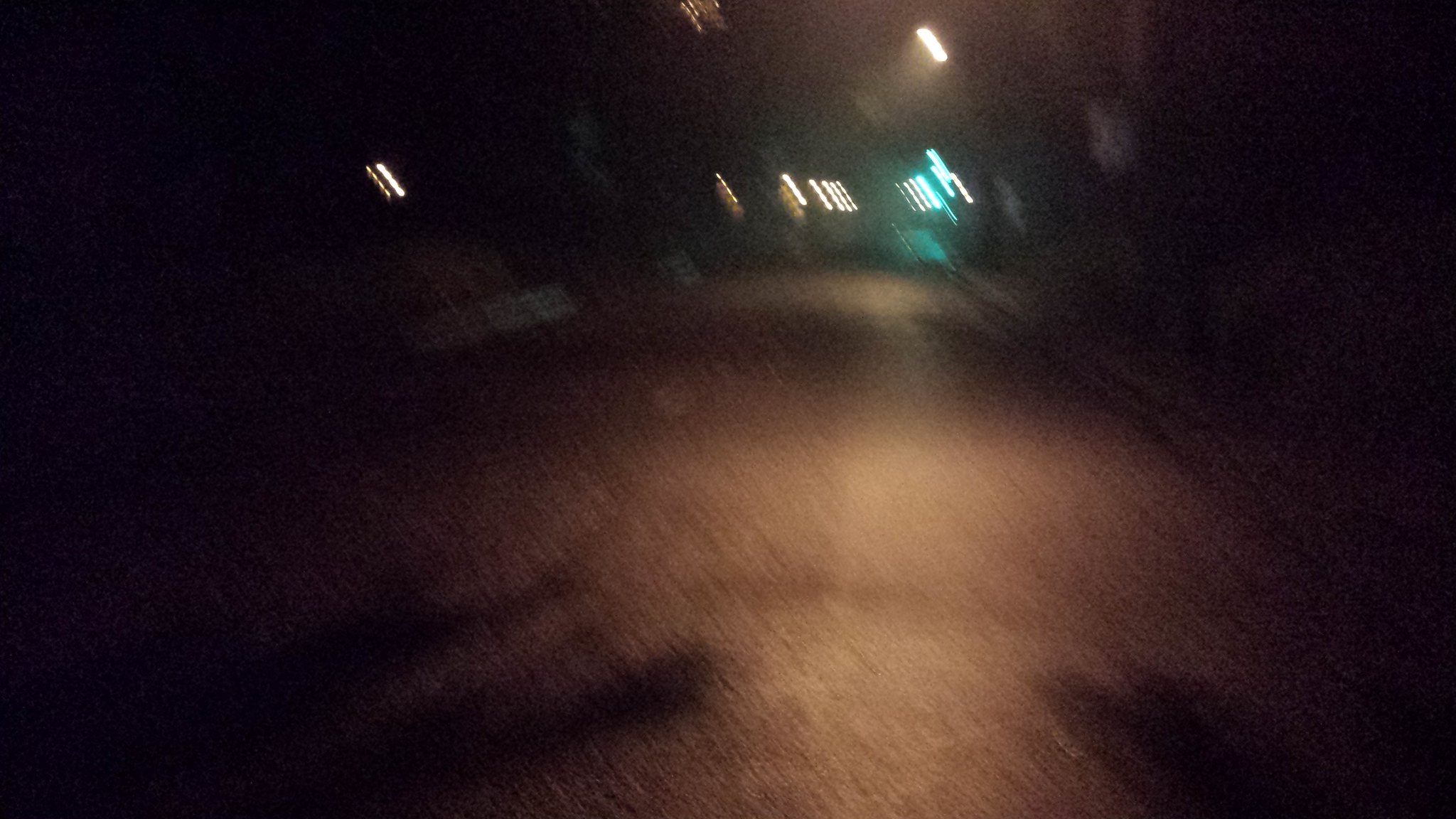This nighttime photograph, although blurry, captures a dimly lit scene. The background is enveloped in darkness, with the faint glow of white and blue-tinted lights visible in the distance. The shot appears to be taken from a straight-ahead angle, likely attached to the photographer, offering a direct perspective. The ground is dark, resembling black concrete, and faint outlines suggest the presence of trees casting shadows upon it. To the side, scattered white lights can be observed, including a distinct rectangular-shaped light that adds a subtle luminance to the murky surroundings.